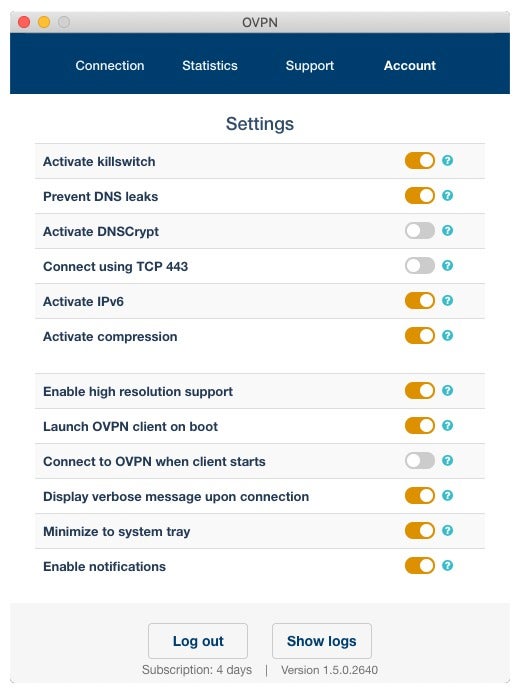This image depicts a user interface of an application running on macOS. The screen features the distinctive macOS gray top taskbar where the highlighted application icon, 'OVPN' in black, uppercase letters, is centered. To the left of this icon are the classic Apple control buttons - red, orange, and gray, which are used to close, minimize, and minimize to the Dock, respectively.

Below the taskbar is a wide, dark blue navigation banner with white text that includes interactive tabs labeled 'Connection', 'Status', 'Support', and 'Account'. These tabs are designed to guide users through different sections of the application.

The main section of the interface is set against a white background with dark blue text, indicating that the 'Settings' menu is currently open. The 'Settings' title is center-aligned at the top of this section. Below, the interface displays several options, each accompanied by an on/off toggle switch. The active toggles are highlighted in orange, while the inactive ones are grayed out. Each setting also has a blue clickable question mark icon for further information.

Toward the bottom of the window, there are two gray buttons with blue text labeled 'Log Out' and 'Show Logs'. Below these buttons, the application's version number is displayed next to an area indicating the number of subscription days remaining. An example of some settings options includes 'Activate Kill Switch', 'Prevent DNS Leaks', 'Enable High-Resolution Support', 'Connect Using TCP 443' (currently grayed out), 'Activate DNSCrypt' (grayed out), and 'Connect to OVPN when client starts' (grayed out).

Additionally, the list of settings options is formatted with alternating shades of gray to improve readability and help users easily match each setting to its corresponding switch. This thoughtful design detail ensures a user-friendly navigation experience.